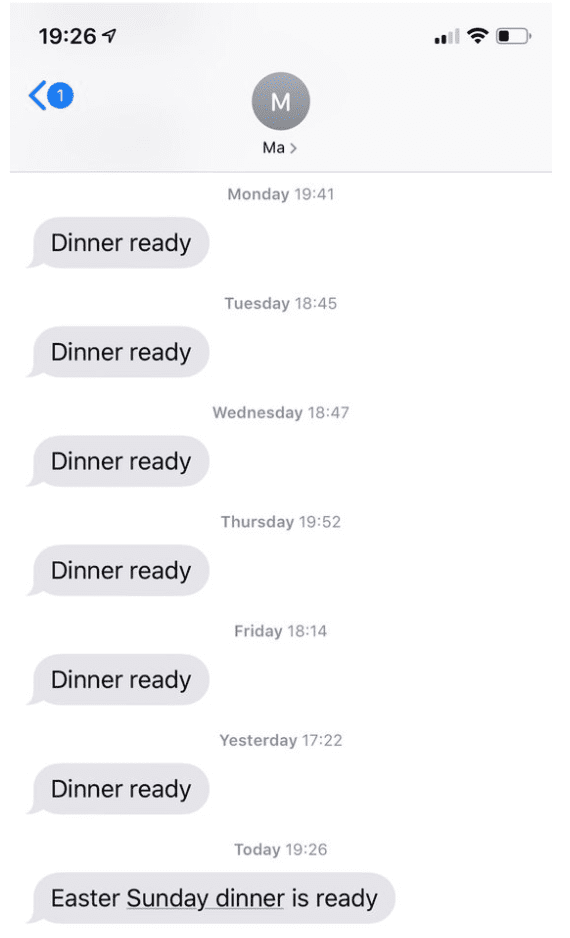The screenshot showcases a series of text messages received on a smartphone. The device's time, displayed in the top-left corner, reads 19:26, indicating it's 7:26 p.m. In the top-right corner, the battery icon shows approximately one-third charge remaining. Near the top, there's a profile picture with a white 'M' on a gray background, identifying the contact as "Ma," presumably the person's mother.

The messages are consistent and routine, each sent around dinner time with variations in exact times. Here's the detailed sequence:

- **Monday, 19:41**: "Dinner ready"
- **Tuesday, 18:45**: "Dinner ready"
- **Wednesday, 18:47**: "Dinner ready"
- **Thursday, 19:52**: "Dinner ready"
- **Friday, 18:14**: "Dinner ready"
- **Yesterday, 17:22**: "Dinner ready"
- **Today, 19:26**: "Easter Sunday dinner ready" or "dinner is ready"

This pattern highlights the mother's consistency in informing her child that dinner is ready, especially noting the special mention of "Easter Sunday dinner" on the current day.